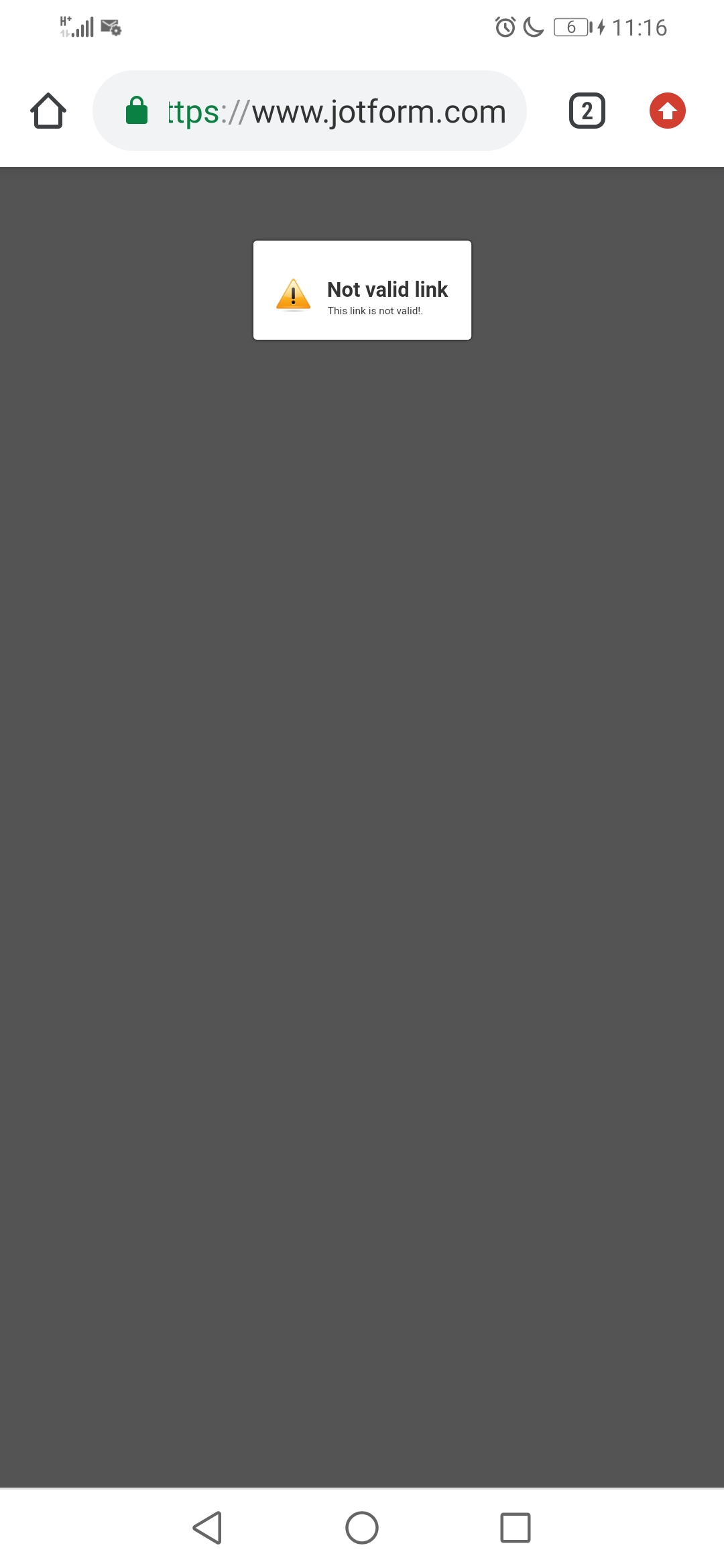This is a detailed screenshot of a mobile phone screen captured while attempting to visit a website. At the very top right corner of the screen, icons are visible, including a battery symbol, a time display showing 11:16, a crescent moon, and a timer. Below these icons, a search bar with a rounded rectangular shape is present, indicating the URL "https://" highlighted in green, followed by "www.jotform.com."

The bulk of the screen, which is meant to display the website's content, appears with a dark gray background. Positioned in the upper-middle right section of this area is a white box containing an orange or yellow caution sign, depicted as a triangle with an exclamation point inside. To the right of this caution symbol, the phrase "Not valid link" is prominently displayed in bold text. Additional text appears below this message, but it is too small to be deciphered.

At the very bottom of the screenshot is the home screen button, indicating this is a navigational element of the phone's interface.